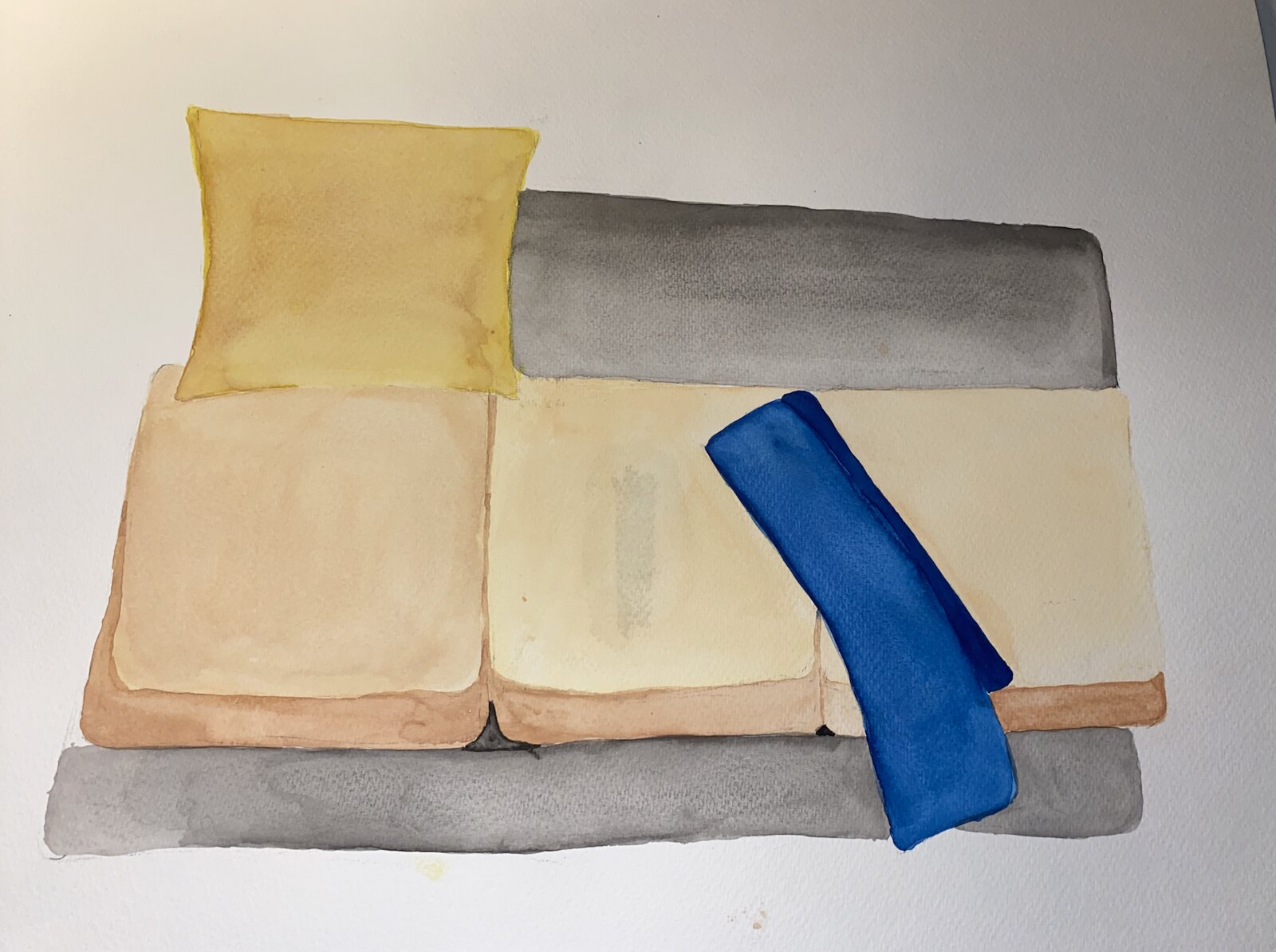This indoor photograph captures a vibrant watercolor painting on white, textured watercolor paper, illuminated by an overhead light source. The texture of the paper is evident, showing through both painted areas and untouched white sections. The top left corner of the image features a pale yellow hue, though it's unclear whether this results from the artwork or the lighting.

The painting itself depicts an abstract representation of a living room setting. Along the bottom of the composition lies a gray rectangle, interpreted as the base of a sofa. Above this, three slightly varied shades of cream and pale brown squares are painted with three-dimensional effect, suggesting sofa cushions. A matching gray shade borders the top of these squares, further defining the sofa's structure.

Dominating the scene is a mustard yellow throw pillow, meticulously rendered with darker and lighter shades of yellow to enhance its depth and three-dimensional appearance. A blue rectangle, which widens slightly as it extends downwards, appears to cascade over the gray form, evocative of a throw blanket draped over the couch. The use of shadow and gradient in color deftly conveys the soft, comforting textures of a cozy living room vignette.